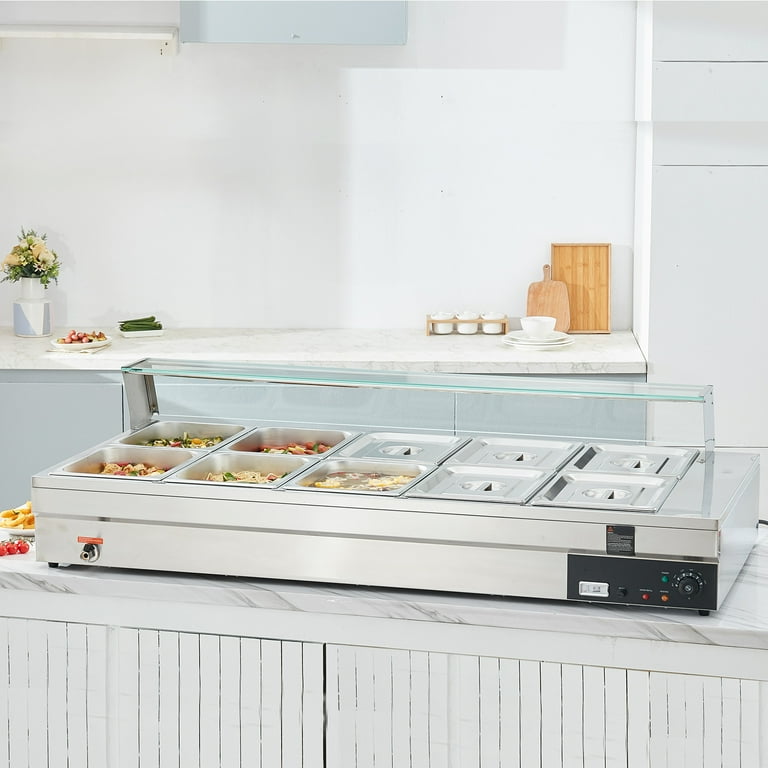This photograph captures a brightly lit breakfast buffet area, possibly in a kitchen or hotel, featuring a prominent white marble countertop in the foreground. Resting on this countertop is a long, sleek food warmer with ten square compartments. The five compartments on the left are open, revealing an array of brightly colored foods with yellow, orange, red, and green bits, although their exact nature is unclear. The remaining five compartments are closed with lids, protected by a glass top sneeze guard, and managed by a control panel featuring a black dial and various buttons on the lower right.

In the background, against a white wall, another marble counter can be seen. This counter is adorned with an eclectic array of items: a vase filled with tan flowers, a white plate bearing a round pink item, another square white plate stacked with long green objects, a cutting board, a tray, and a stack of plates with a bowl on top. Additionally, there are three white canisters placed inside a wooden holder, completing the scene.